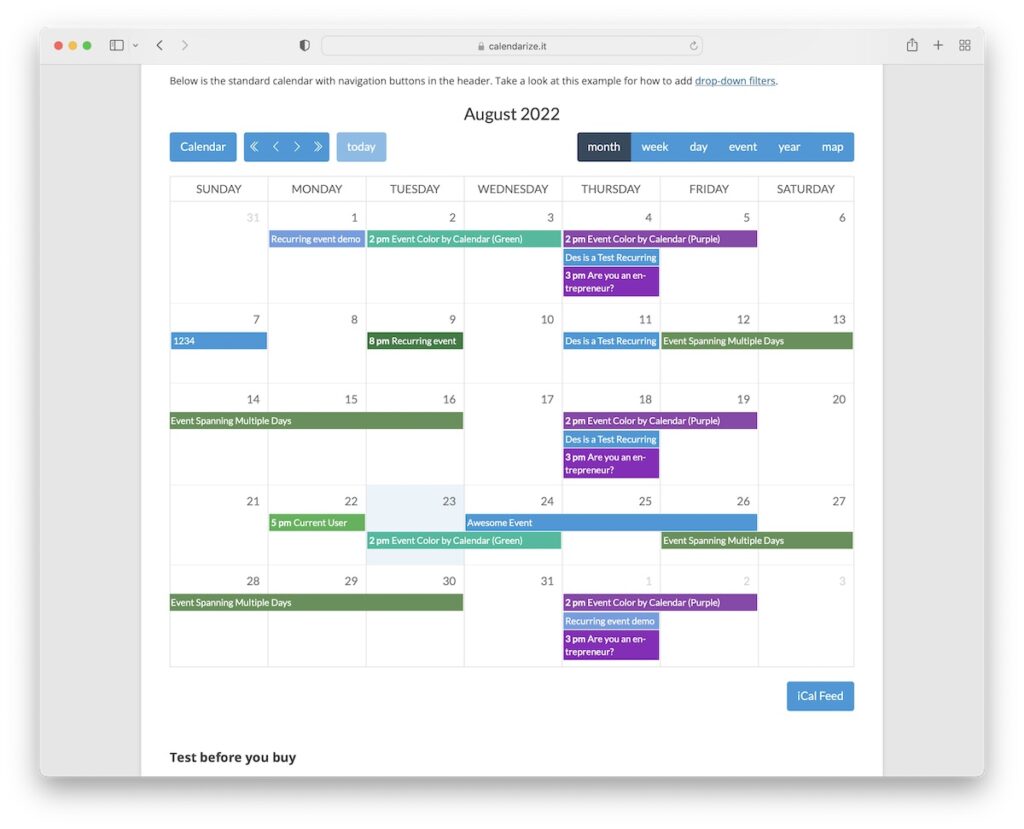**Detailed Descriptive Caption of Calendar Interface on Apple MacBook:**

The image showcases a detailed view of a calendar displayed on an Apple MacBook. The distinct dark gray bezel and the characteristic three circles—red, orange, and green—on the left confirm the device's identity as a MacBook. Positioned slightly right of center is a URL accompanied by a shield icon, divided half black and half white, and a gray padlock, signifying a secure connection.

In the calendar application, the interface is primarily white, featuring black text that reads: "Below is a standard calendar with navigation buttons in the header. Take a look at the example for now." Additionally, a blue hyperlink text states "drop down filters." The current month, "August 2022," is prominently displayed in bold black text.

On the left side, the interface includes several dark blue navigation buttons with white text and symbols: double arrow to the left, single arrow to the left, single arrow to the right, and double arrow to the right. There is also a light blue button labeled "Today" with white text.

Adjacent to "August 2022," a selected button in dark blue reads "Month" in white, indicating the view mode. Other view mode options displayed in mid-blue with white text include Week, Day, Event, Year, and Map.

Events are color-coded on the calendar using dark blue, teal green, cyan blue, and purple for better visual distinction. Starting with Monday, there is a dark blue rectangle noting "Recurring Event Demo" in white. On Tuesday at 2 p.m., a green rectangle marks "Event Color Calendar (Green)."

From Thursday to Friday, a purple rectangle spans the days, highlighting "2 p.m. Event Color by Calendar (Purple)." Thursday also contains additional events like "Death is a Test Recurring" in a blue rectangle and "3 p.m. Are You?" in a purple rectangle.

On Sunday the 7th, a dark blue rectangle reads "1 2 3 4" in white. Then, from Thursday the 8th to the 9th, a green rectangle shows "8 p.m. Recurring Event." On Thursday the 11th, a blue rectangle states "Death is a Test Recurring," followed by a dark green rectangle from the 12th to the 13th noting "Event Spanning Multiple Days."

From the 14th to the 16th, the same dark green rectangle continues with the statement "Event Spanning Multiple Days." On the 18th and into the 19th, a purple event note reads "2 p.m. Event Color by Calendar (Purple)," followed by another purple rectangle at 3 p.m. stating "Are You an Entrepreneur."

On the 22nd, a light blue or green rectangle at 5 p.m. notes "Current User" in white. An event on the 23rd is indicated by a teal rectangle labeled "2 p.m. Event Color by Calendar (Green)." From the 24th to the 26th, a dark blue rectangle highlights an "Awesome Event" in white.

The period from the 26th to the 30th features a dark green rectangle stating "Event Spanning Multiple Days" in white. On the first of the next month, a purple rectangle marks "2 p.m. Event Color by Calendar (Purple)," followed by another dark blue rectangle at 2:45 reading "Recurring Event Demo" in white. On the same day, a large purple rectangle at 3 p.m. notes "Are You an Entrepreneur."

At the bottom right of the interface, a button labeled "iCalsFeed" (with a lowercase 'i' and capital 'C' and 'F') appears. On the lower left side, bold black text reads: "Test Before You Buy."